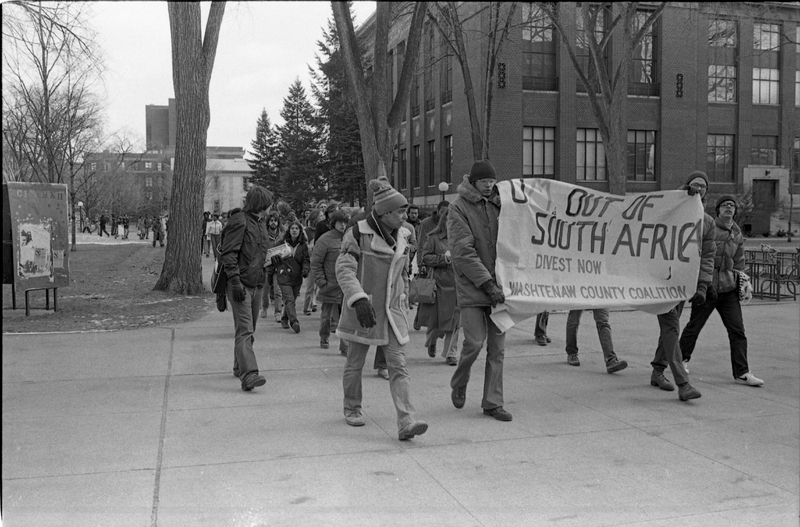This vintage black and white photograph captures a significant protest from what appears to be the late 60s to mid 70s, set against the backdrop of a college campus or possibly a GM plant, evidenced by the mention of 'GM' on a prominent banner. The scene portrays a large line of relatively young people, dressed warmly in winter coats, gloves, and toboggans, marching in unison on a cold day. Leading the charge are several men holding a large white poster emblazoned with the plea “GM out of South Africa, Divest Now, Washtenaw County Coalition.” The marchers proceed along a pathway flanked by buildings with large glass windows, recognizable as campus or industrial structures, and interspersed with bare trees. The background includes a directory sign and various structures, indicating an organized and well-attended demonstration, rallying for divestment and social change during a turbulent period.